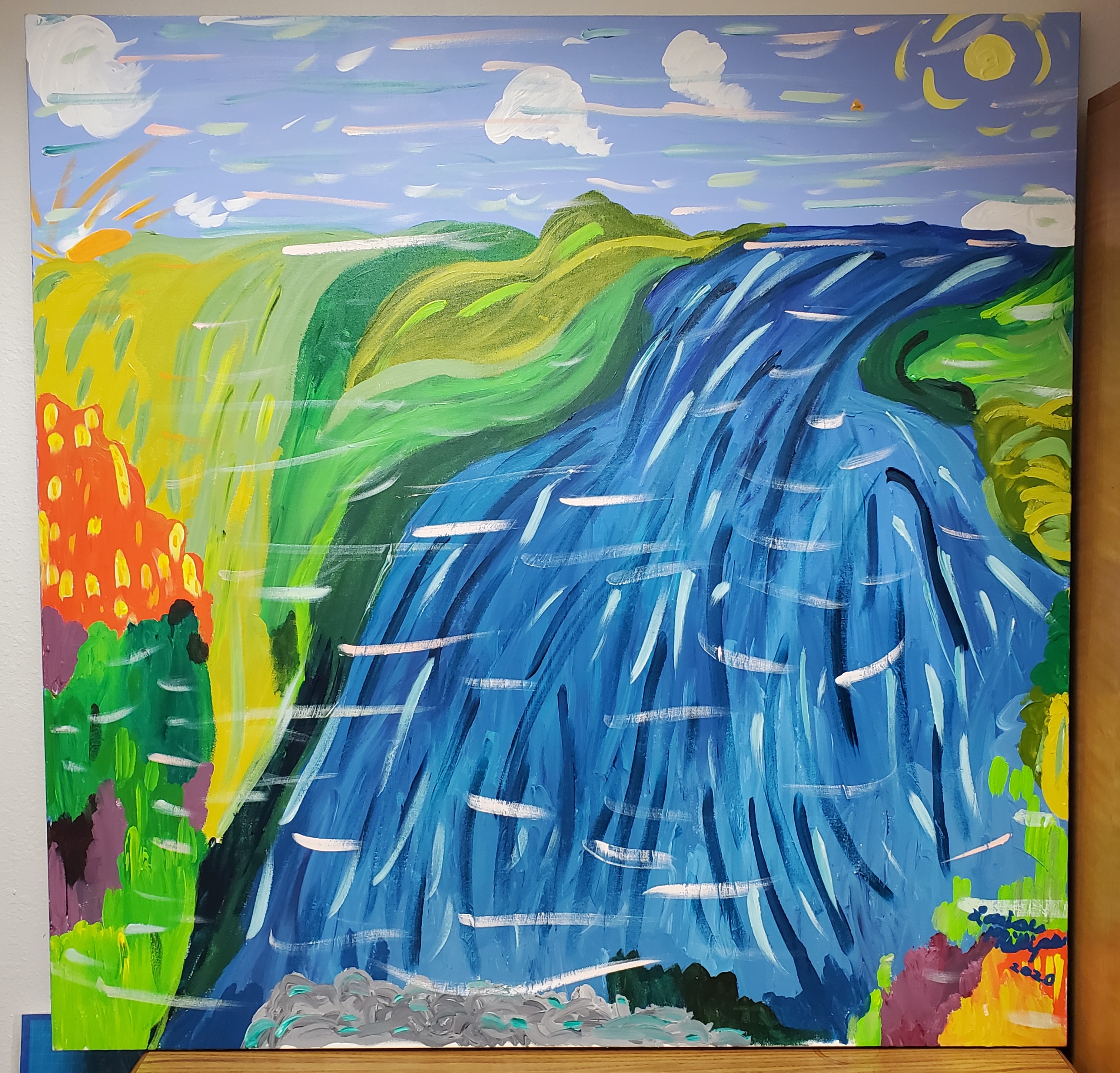This painting, likely created by an amateur artist, depicts a vivid, albeit simplistic, waterfall scene. At the top of the canvas, a light blue sky is rendered with white clouds, including a prominent one on the far left, one in the middle, and a smaller one to the right, along with a radiant yellow sun in the top right corner. Some descriptions also mention a second orange sun in the left corner, adding an abstract element to the composition.

The waterfall itself is the central focus, beginning slightly to the right and cascading down to the bottom of the canvas. The water flow is characterized by a large blue area and meets a pool of water decorated with gray, white, and teal hues, suggesting the splashing water at the base. Surrounding the waterfall, varying shades of green depict lush greenery, which includes areas of grass, flowers, and bushes on both sides. Notably, red and purple flowers can be seen amidst the greenery. Additionally, an orange tree with yellow flowers contributes to the vibrant palette of the scene.

The painting features broad paint streaks, indicating a chosen stylistic approach that lends a child-like simplicity to the overall composition. Despite its rudimentary execution, the painting's use of colors such as blue, green, yellow, orange, purple, and gray creates a lively and feel-good atmosphere. The artist's signature and the year 2020 are inscribed on the bottom right corner, cementing the artwork as a unique and personal expression.